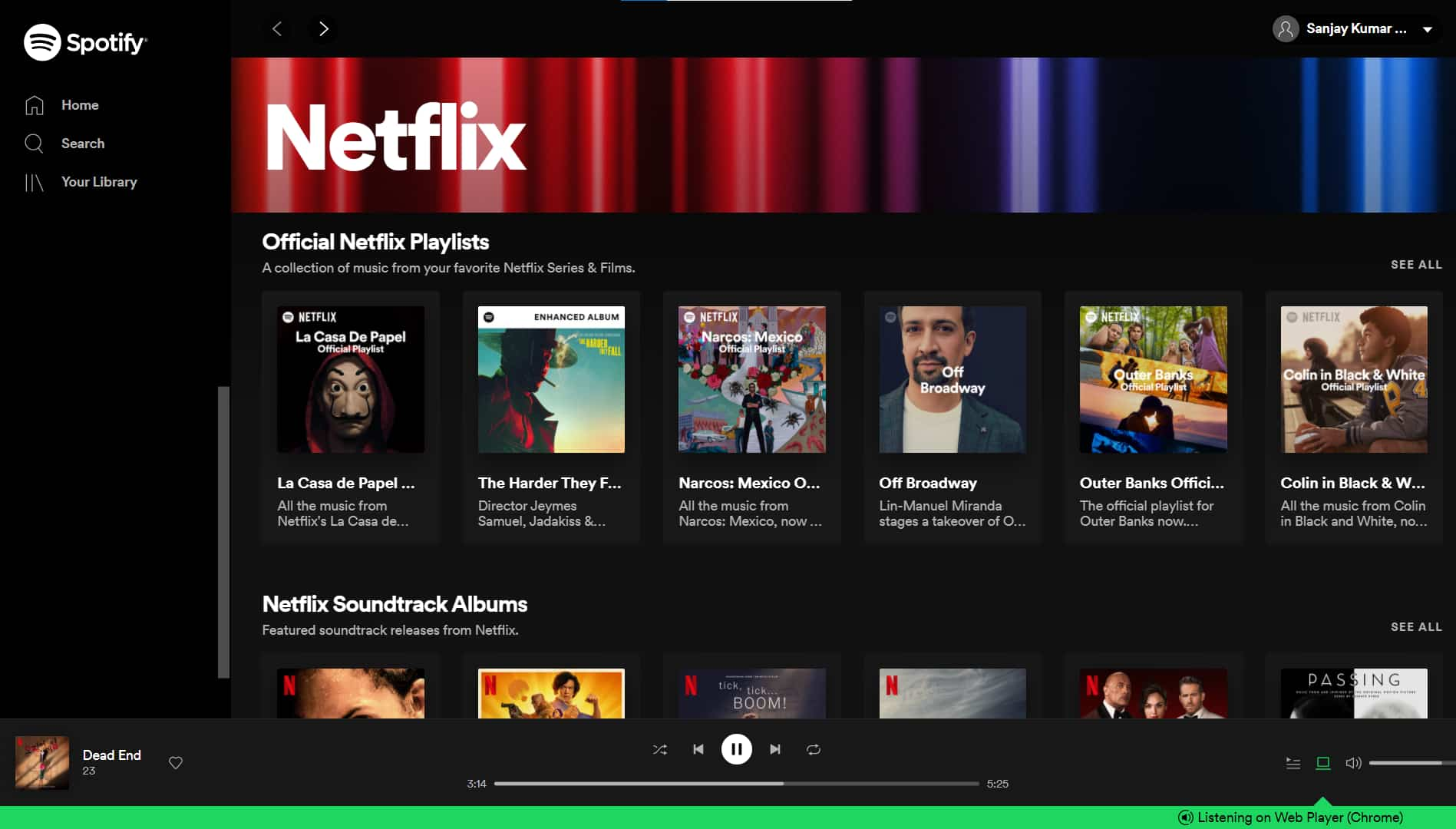The image depicts a Spotify interface with a banner promoting Netflix playlists. The background is predominantly solid black. In the upper left corner, the white Spotify logo and the word "Spotify" are prominently displayed. Down the left side of the interface, there are three navigation options: a home icon labeled "Home," a magnifying glass icon labeled "Search," and a book icon labeled "Your Library."

To the right of these options, a large banner showcases the word "Netflix" in white letters, set against a background of vertical bars transitioning in color from red to purple to blue, and finally to a lighter blue on the far right. Beneath this banner, smaller white text reads "Official Netflix Playlists" and "A collection of music from your favorite Netflix series and films."

Central to the page, six horizontally aligned boxes each contain images representing different playlists. Below each image are titles and two lines of descriptive text.

Near the bottom of the image, the text "Netflix Soundtrack Albums" appears, followed by another row of six images. However, only the tops of these boxes are visible.